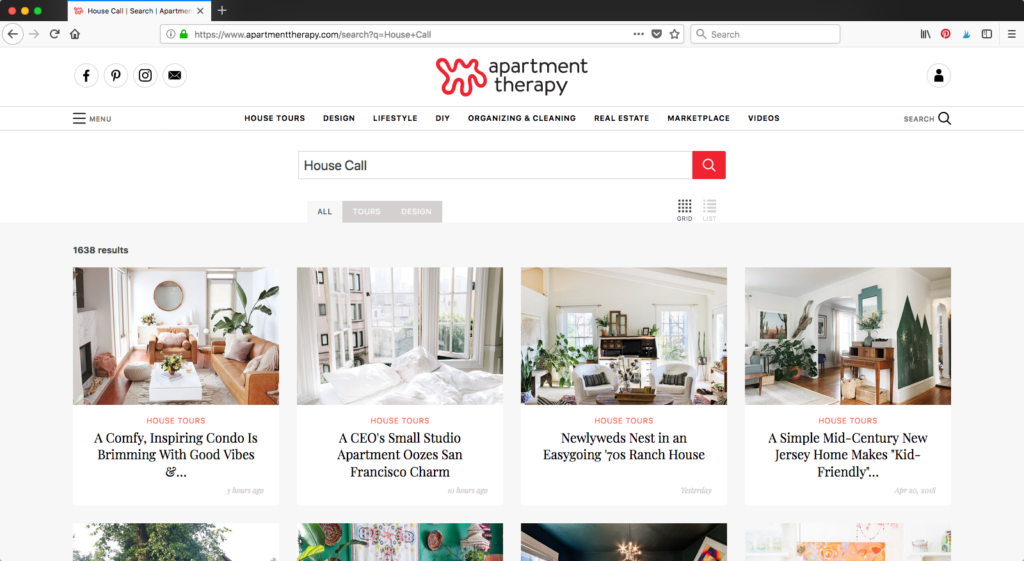The image depicts a webpage displayed on the Safari browser, identifiable by the red, yellow, and green circles in the upper left corner. The URL at the top reads "www.apartmenttherapy.com," indicating that the site belongs to Apartment Therapy. The logo features a unique red outline resembling a track or course, situated next to the text "Apartment Therapy."

On the left side of the page, social media links for Facebook, Pinterest, and Instagram are visible. To the right, there are icons for user login, a menu (denoted by three horizontal bars), followed by navigation links labeled: House Tours, Design, Lifestyle, DIY, Organizing & Cleaning, Real Estate, Marketplace, Videos, and a search icon.

Below this navigation bar is a search box with "house call" inputted and a red search button. The search results display a total of 1,638 entries, showcasing various interior designs from different homes. One example highlighted is titled "A Comfy Inspiring Condo is Brimming with Good Vibes," featuring an image of a clean, beautifully furnished white living room. Four similar interior thumbnails are visible, while the rest are cut off.

The overall design of the website is minimalistic with a white background, black text, and occasional red accents, primarily around the search button and logo.